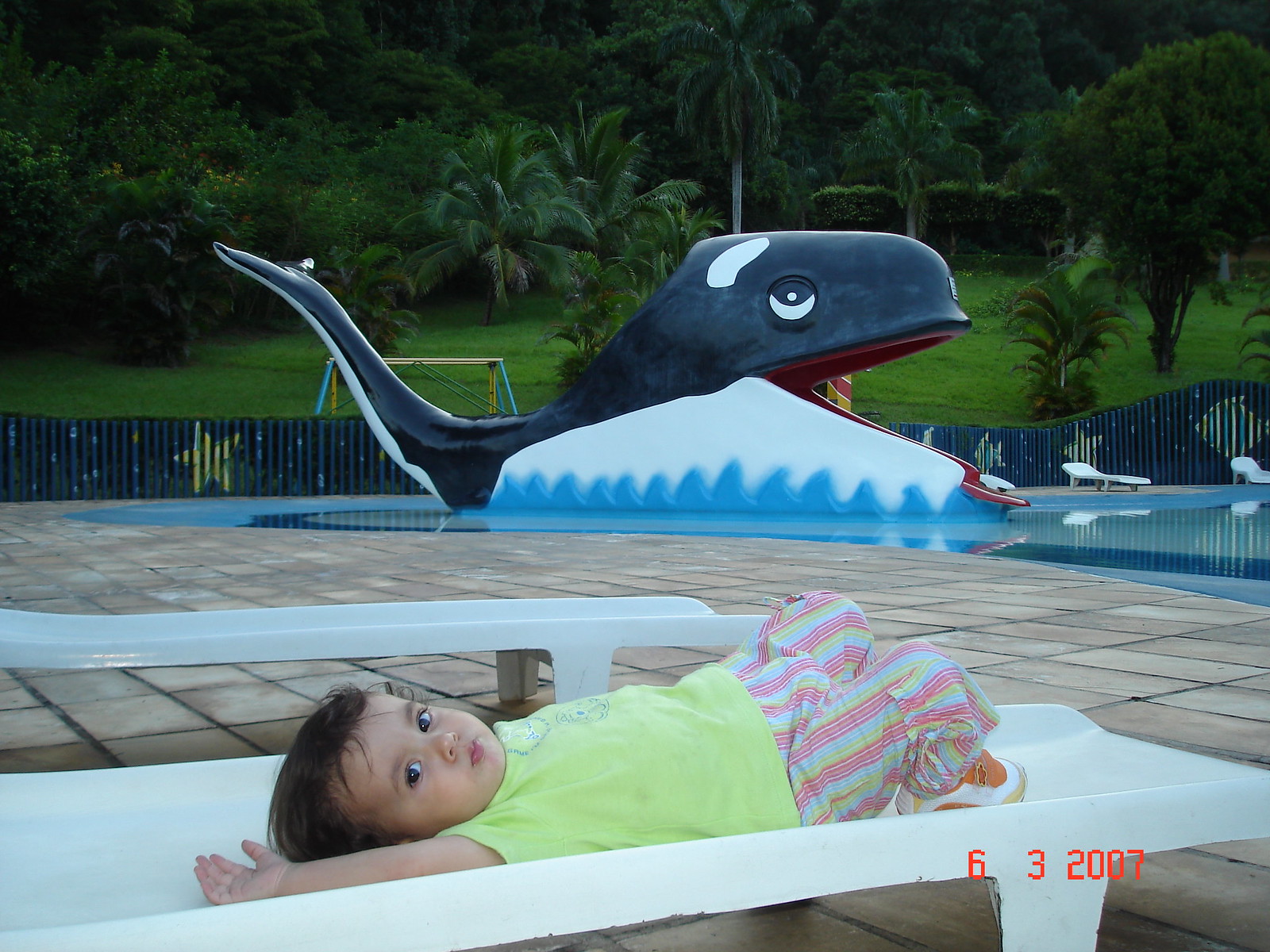In this photograph taken on 6-3-2007, a baby is lounging on a low-riding white plastic deck chair by a pool. The baby, dressed in a yellow t-shirt and colorful pajama bottoms, has their hands behind their head and looks directly into the camera. The pool area is adorned with brown rectangular tiles and features a striking black and white whale slide. Beyond the pool's blue fence, which is decorated with stars and fish, there is an expanse of green grass and palm trees, suggesting a Florida location. In the distant background, a yellow and blue swing set is partially visible, framed by tall hedges. The serene and playful setting captures a moment of relaxation and fun.